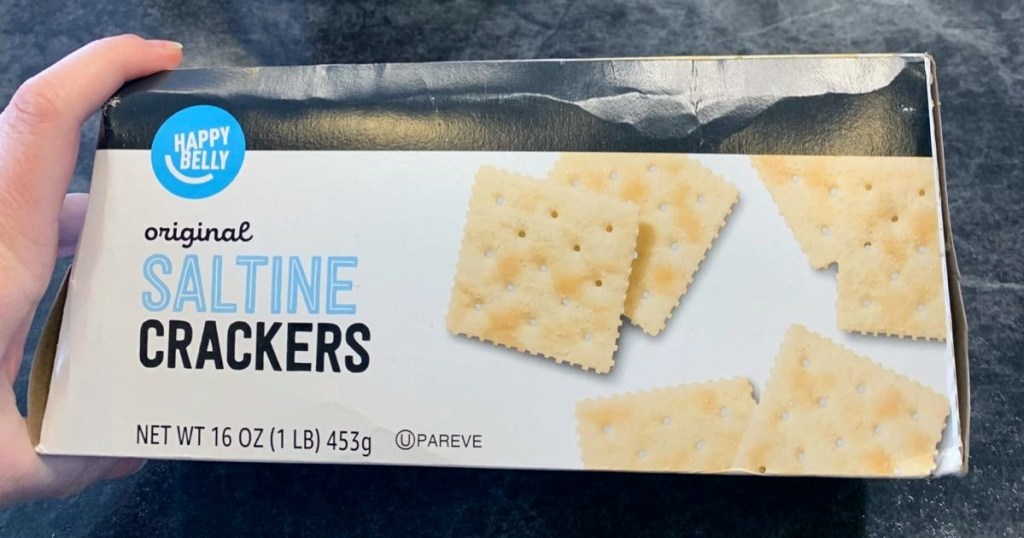The image portrays a box of Happy Belly Original Saltine Crackers positioned against a dark, cloud-like gray background that mimics a decorative countertop design. A person's left hand, belonging to a white individual, is holding the box with their index finger and thumb. The rectangular box, occupying the majority of this landscape-oriented photo, is predominantly white with a horizontal black stripe at the top. Within this stripe, on the upper left, is a light blue circle with white text reading "Happy Belly." Below it, written in a small cursive black font, is the word "original." Further down, the words "saltine" and "crackers" appear in blue and black text, respectively. Additional details include the net weight of 16 ounces (1 pound or 453 grams) and a certification symbol - a 'U' within a circle, alongside the word "PAREVE." On the right side of the box, the illustration shows several saltine crackers arranged in overlapping groups of two. The setting of the photo suggests it was taken in a kitchen, with the hand holding the product prominently in the lower left foreground.